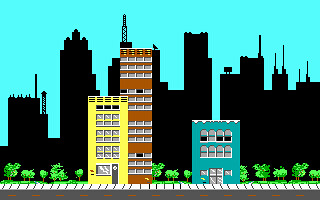This small square digital image from a retro-style video game depicts a simplified cityscape with vibrant colors and geometric shapes. In the foreground, there is a gray road with little orange lines, flanked by a white sidewalk and neat green shrubbery. Beyond this, three distinct buildings stand prominently. To the left, a four-story yellow building with vertical rectangular windows is connected to a taller, narrower brown building with horizontal rectangular windows. Both buildings share a single door on the yellow section. Spaced slightly apart to the right, there is a three-story blue building with double doors at the bottom and rounded windows forming two rows at the top. Behind these structures, a line of trees stretches from left to right. In the distant background, the silhouettes of around ten black skyscrapers, adorned with various antennas and towers, rise against a solid light blue sky, completing the simple yet detailed urban scene.